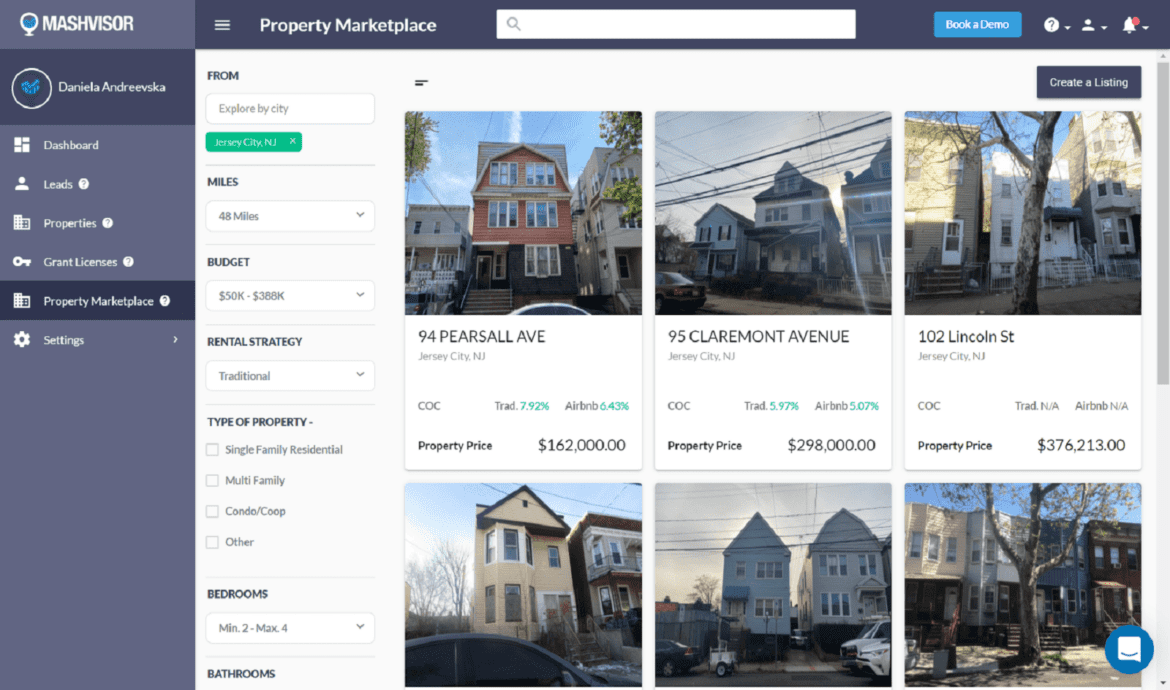This image displays the interface of Mashvisor, a property marketplace website that aids users in finding and investing in real estate. The site allows users to explore listings by entering specific criteria such as city, distance from the user’s location, budget, rental strategy, and property type. This screenshot particularly showcases a search for rental properties in Jersey City, New Jersey, with the rental strategy set to "traditional" and a focus on single-family homes. Property prices on the displayed page range from $162,000 to $376,000, indicating a selection of investment opportunities where users can purchase properties to rent out. The dashboard provides a comprehensive and user-friendly tool for potential real estate investors to navigate through available listings tailored to their investment goals.